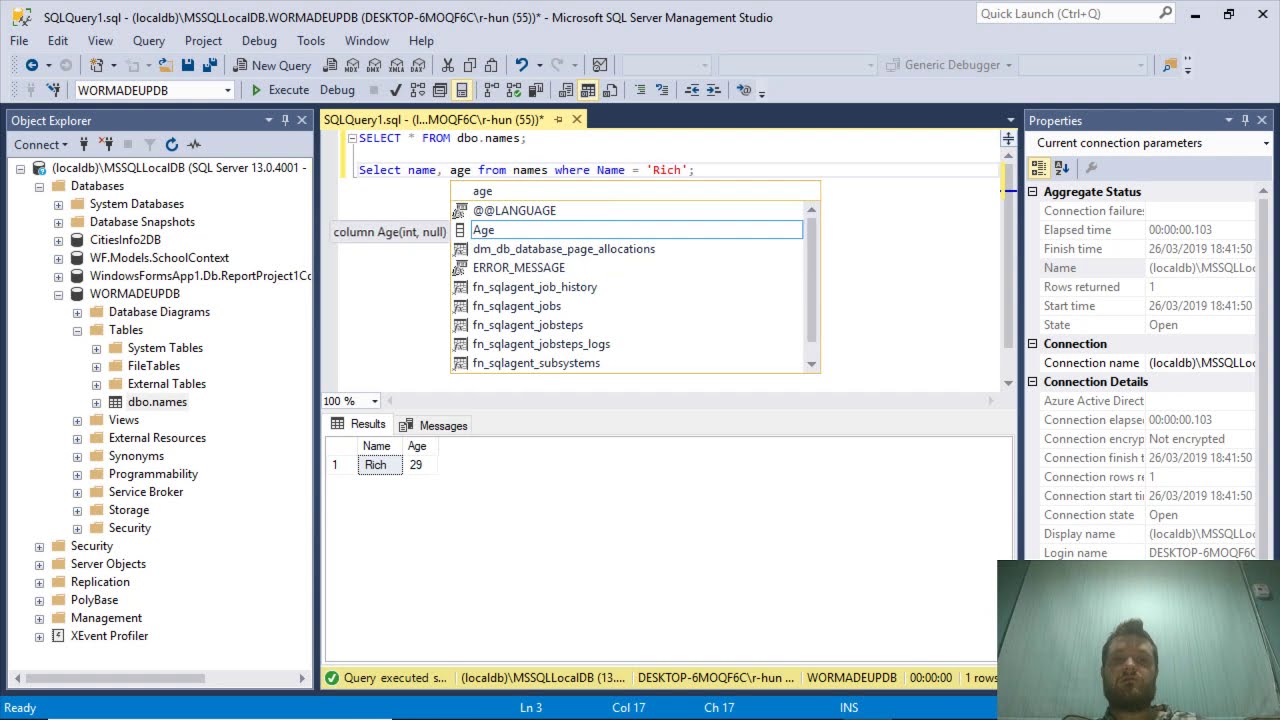The image displays a detailed snapshot of a computer screen with a multi-panel interface used for database management and SQL queries. The interface is divided into three columns. The leftmost column at the top is titled "opt," containing a list of database-related files, including "system databases" and "snapshots." In the center column, labeled "SQL QE," a section labeled "age" is visible, followed by a result indicating a single row: "Number one, Rich, age 29." The rightmost column provides details on current connection parameters, displaying properties such as "aggregate status."

The interface features a blue toolbar with various options including File, Edit, View, Query, Project, Debug, Tools, Window, and Help. At the top, the header reads "SQL Query" in prominent black text on a gray background. Throughout the screen, various document and file folders can be seen, each containing numerous files that are difficult to read due to their small size, with some recognizable words such as "language," "age," and "error message."

In the bottom right-hand corner of the screen, there's a small video thumbnail showing a Caucasian gentleman with short brown hair and a full gray beard, against a background of a whiteboard and a white wall. This thumbnail appears to be a live or recorded view of the person currently using the computer, viewed from a low-angle perspective.